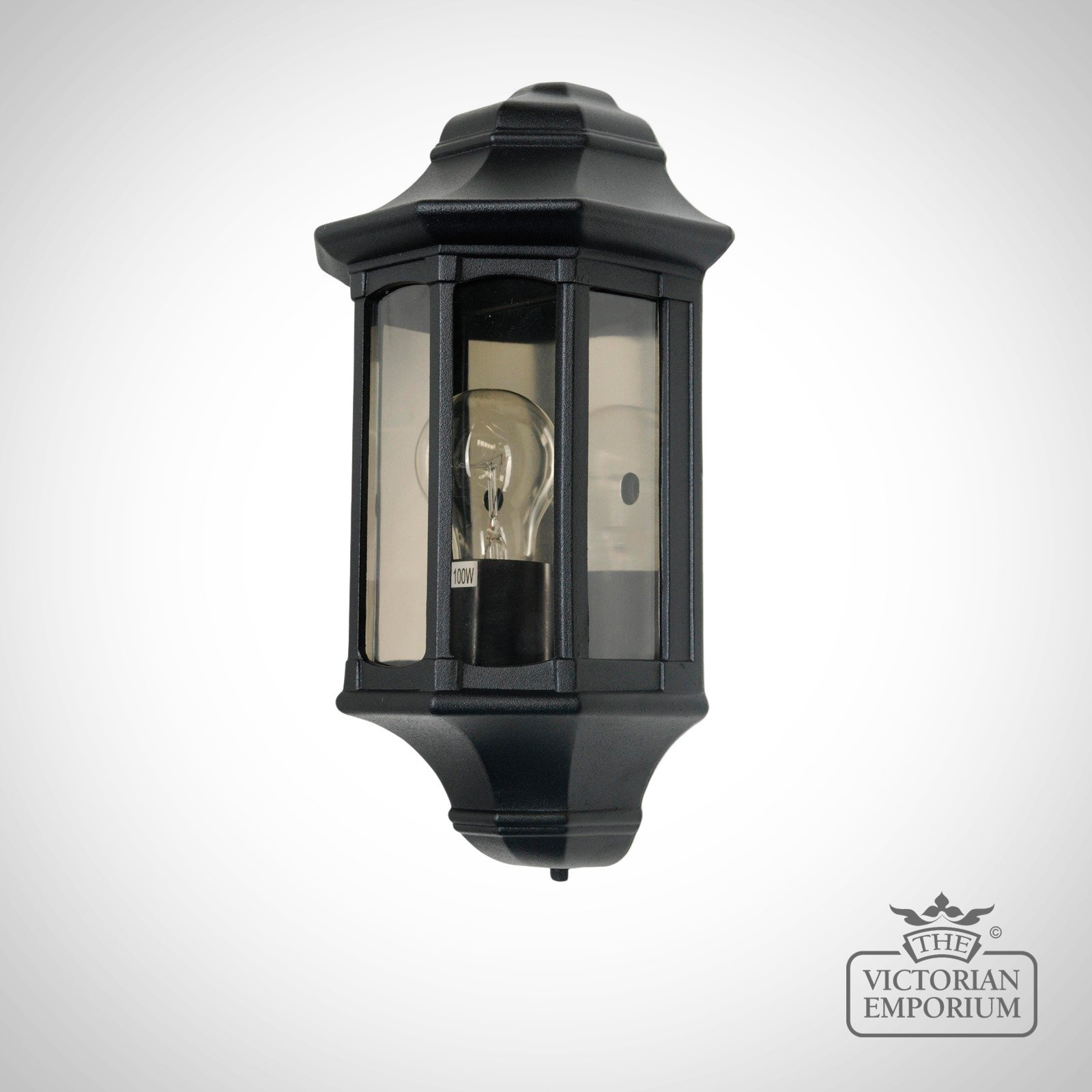The image features an antique-style wall-mounted lamp with a distinct, black, hexagonal design, reminiscent of an old-fashioned streetlight. The lamp comprises a black outer frame forming a three-dimensional hexagonal shape, encasing three clear glass panels that slightly yellow with age. These panels are divided by black borders, revealing an unlit, traditionally shaped light bulb, secured on a black base within the fixture. 

The background is predominantly white, fading to a light gray toward the corners. A decorative emblem graces the bottom right corner, featuring three interconnected triangles and an ornate floral design. Adjacent to this emblem, a gray rectangle with the black-outlined text "The Victorian Emporium" stands out, anchoring the antique aesthetic of the piece.